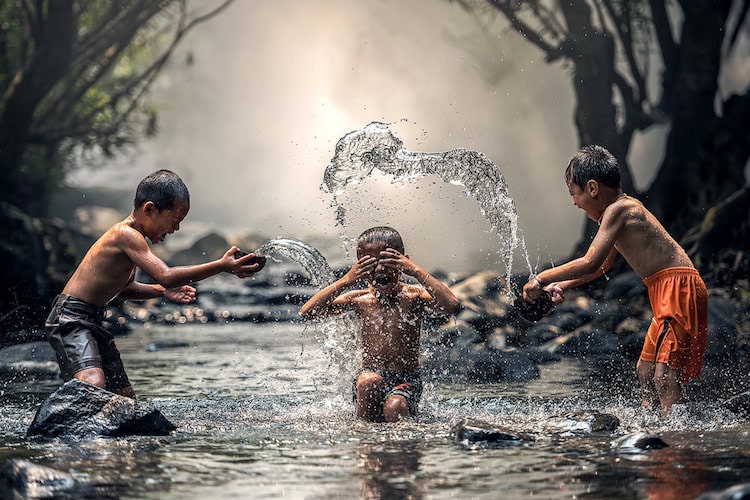In this captivating image, three young boys are energetically playing in a small stream surrounded by a misty, wooded area. The lush, dark trees along the rocky banks arch towards each other, creating a natural canopy that adds to the enchanting atmosphere. The boy on the left, dressed in black shorts, is leaning forward with his drenched hair, about to splash water towards the center. In the middle, the second boy, whose trunks are partially visible, is laughing heartily with his eyes covered to shield himself from the incoming torrent of water. On the right, the third boy, wearing orange shorts, is joyfully splashing water at the central child. All three boys have short hair and their reflections shimmer on the water's surface. A significant splash of water is seen cascading over the boy in the center, perfectly capturing their playful moment amidst the serene and slightly foggy backdrop.